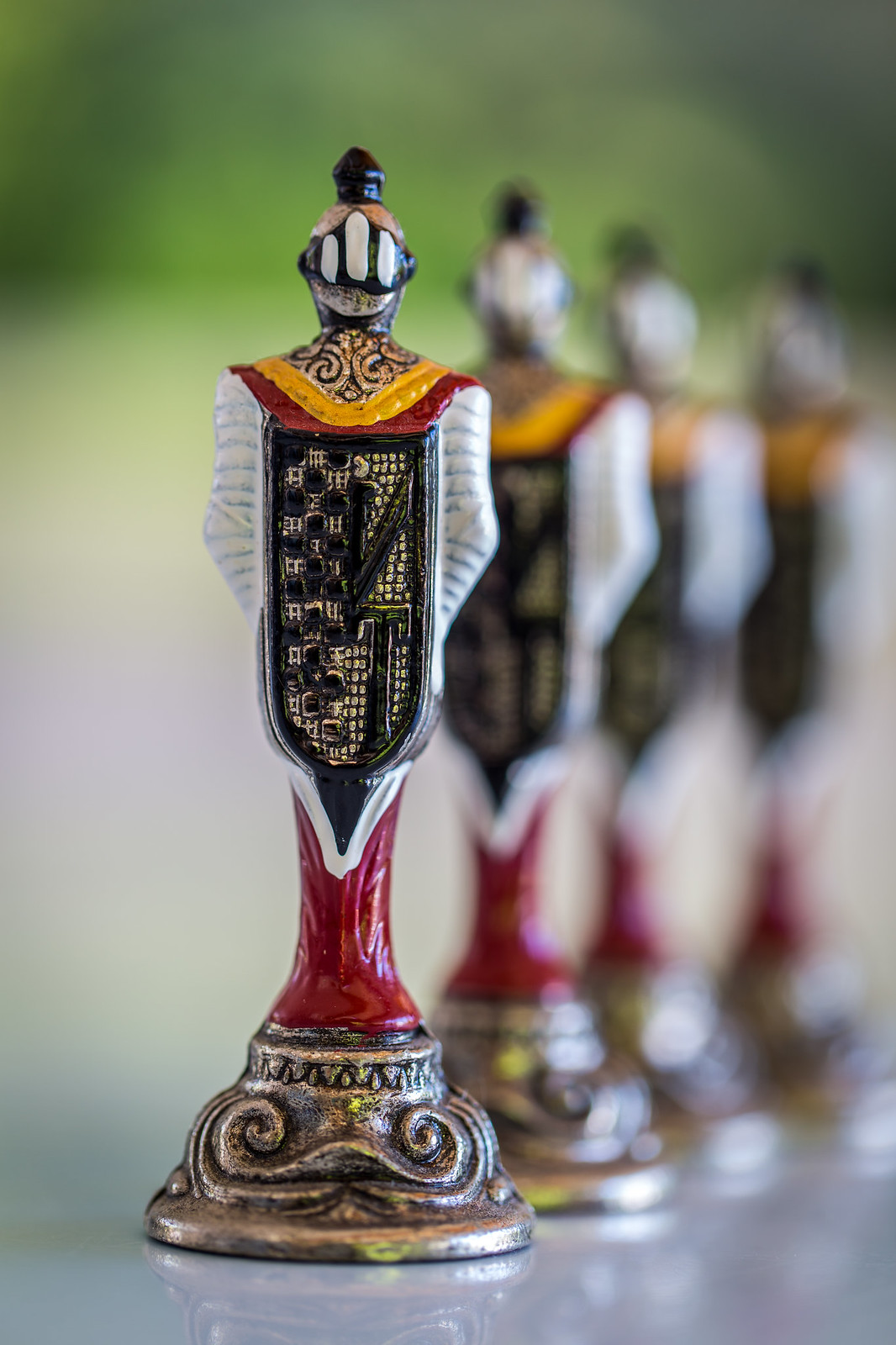The image depicts four intricately detailed knight figurines, possibly chess pieces, arranged in a row. The photograph, taken indoors with a blurred background, emphasizes the foremost piece, which is captured in sharp focus. Each knight is adorned in elaborate armor with a helmet, shield on the chest, and a red, yellow, and gold garment around the neck. Their hands rest at their sides, and they stand atop brass-colored bases adorned with designs. The brave knight in the foreground stands out due to its crisp clarity, with the rest fading softly into the background. The finely detailed front figure showcases the high resolution of the image, revealing every intricate design of the knight's adornments.